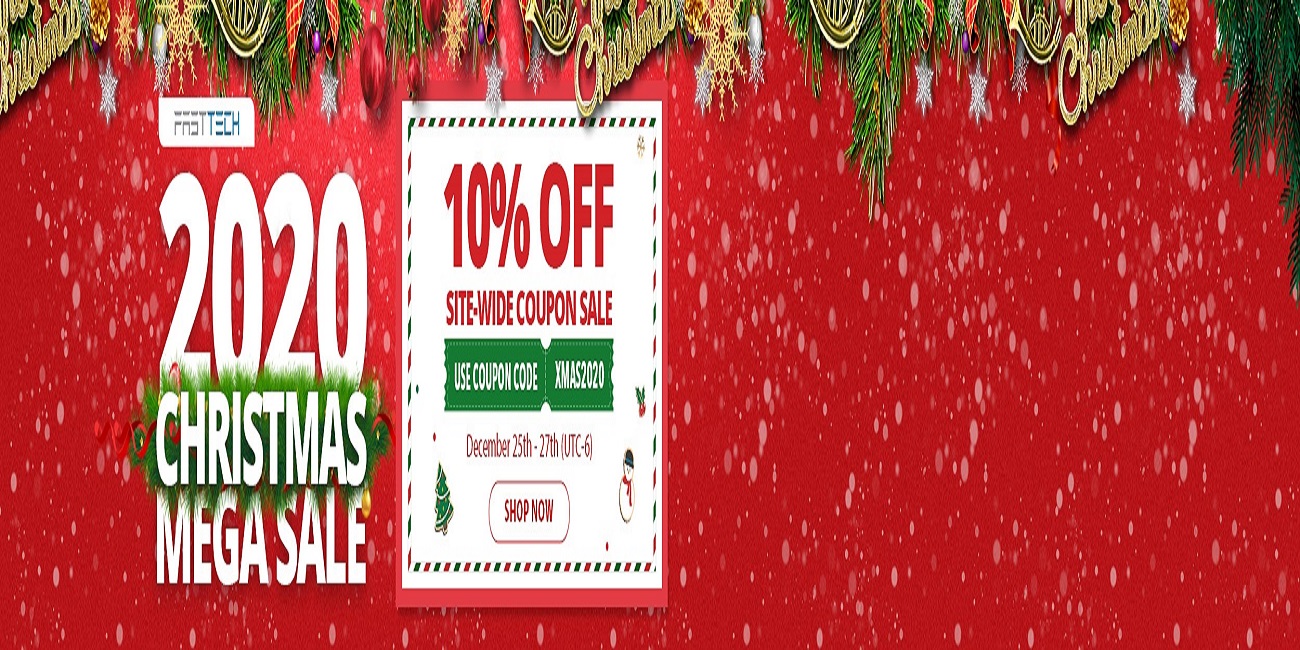The advertisement is for a Christmas sale with a festive red background adorned with falling white snowflakes, depicted as translucent circles. At the top of the image, there's a beautifully decorated Christmas tree surrounded by falling leaves, a gold "Merry Christmas" sign, and a mix of snowflake, red, and purple ornaments, creating a repeating pattern from the top left to the top right.

On the left side of the image, "Fast Tech 2020 Christmas Mega Sale" is prominently displayed in large white letters, with the word "Christmas" set against a decorative wreath background. On the right side, a postcard graphic announces a "10% off sitewide coupon sale" in bold red text. Below this, there is a green ticket with the instructions "Use Coupon Code XMAS2020" displayed in white letters. Further down, details of the sale are provided in red text, stating, "December 25th to 27th UTC-6," and a "Shop Now" button is invitingly placed underneath.

The image is accented with a Christmas tree icon on the left and a snowman with a mistletoe above it on the right, enhancing the overall festive atmosphere of the advertisement.